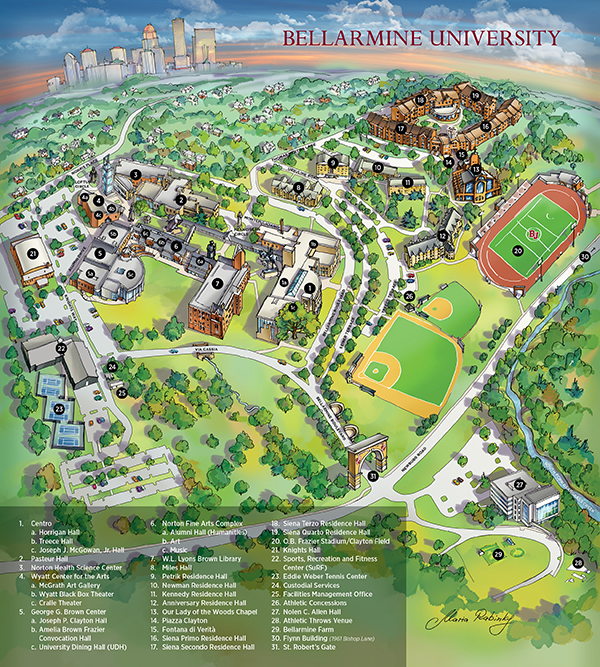This animated map of Bellarmine University, prominently labeled in red in the upper right-hand corner, presents a detailed and stylized aerial view of the campus. The background features a blue sky dotted with white clouds and an orange-pink horizon line, creating a colorful and engaging visual. In the upper left corner, there's an artistic depiction of a cityscape with tall buildings, showcasing a mix of red, peach, tan, white, and brown rooftops.

The central portion of the map is dominated by various university buildings and housing developments, each color-coded with different roofs and labeled with black circles containing white numbers. A detailed legend at the bottom of the map, set against a gray background and numbered 1 through 31, identifies the names of all the halls, chapels, and other significant buildings.

Additional campus features include green and orange baseball diamonds, a football field with a reddish track surrounding a green field marked by white lines, and multiple tennis courts. Abundant trees and lush greenery add to the map’s natural charm. 

In the bottom left corner, a dark transparent rectangle with white text provides further information, including a signature that appears to read "Gloria Robinski." This cartoony, globe-like illustration serves as an inviting guide for visitors navigating the Bellarmine University campus.